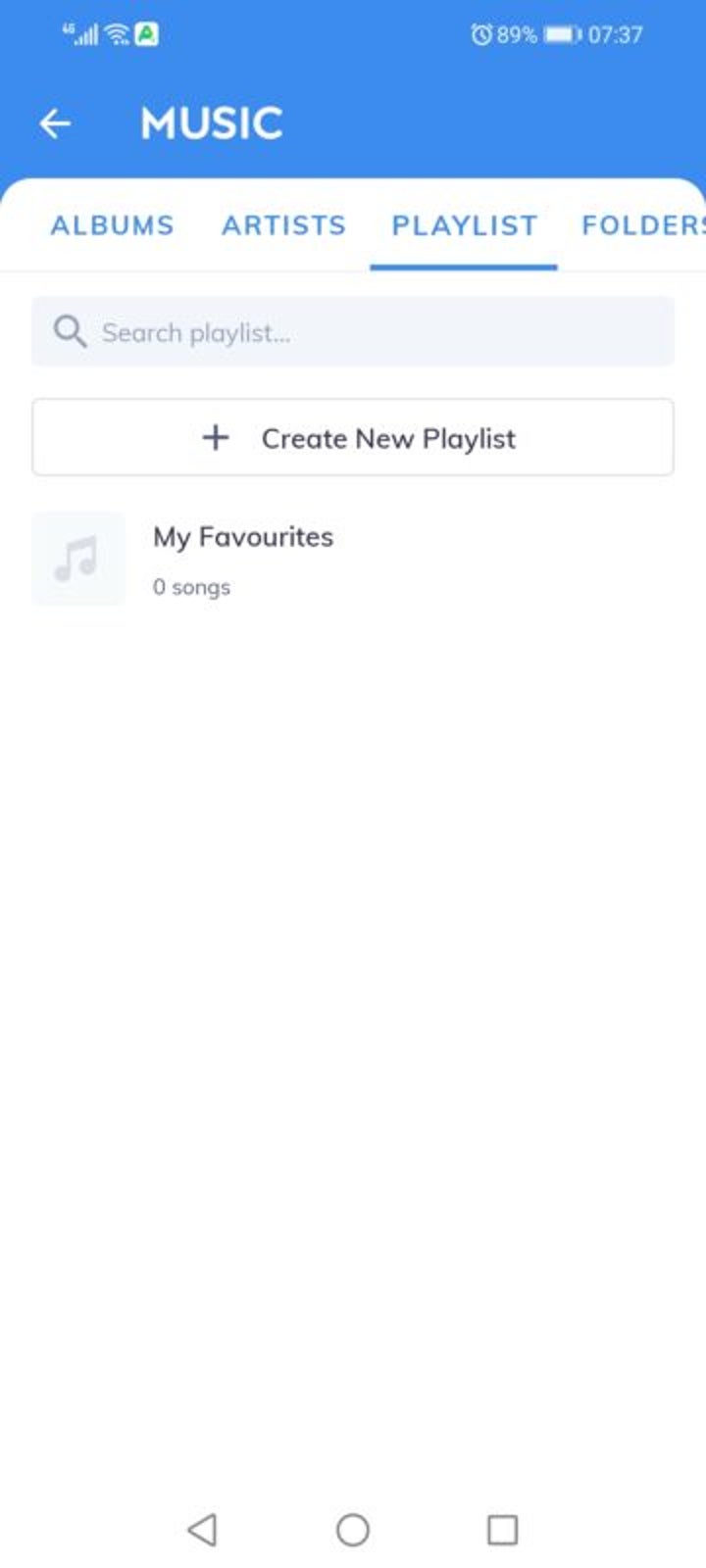This is a detailed screenshot of a cell phone's music application interface. At the top of the screen, various icons indicate the phone's status, including an alarm clock symbol, a battery icon showing 89% charge, and the current time displayed as 7:37. Below these icons, a navigation arrow points left, followed by the label "Music."

The interface features navigation tabs labeled "Albums," "Artists," "Playlists" (which is underlined to denote the current selection), and "Folders." A search bar is situated below these tabs, containing a magnifying glass icon and the prompt "Search playlists."

Further down, there is a black plus sign along with the text "Create new playlist." Adjacent to this, a gray square containing a dark gray music note icon is displayed, accompanied by the text "My Favourites," spelled in British English (F-A-V-O-U-R-I-T-E-S), indicating zero songs in the playlist.

At the bottom of the screen, there are three navigation icons: an arrow pointing left, a circle, and a square. The overall image is portrait-oriented, taller than it is wide, and entirely graphical with no photographic elements or illustrations of people, animals, plants, vehicles, or any other objects.